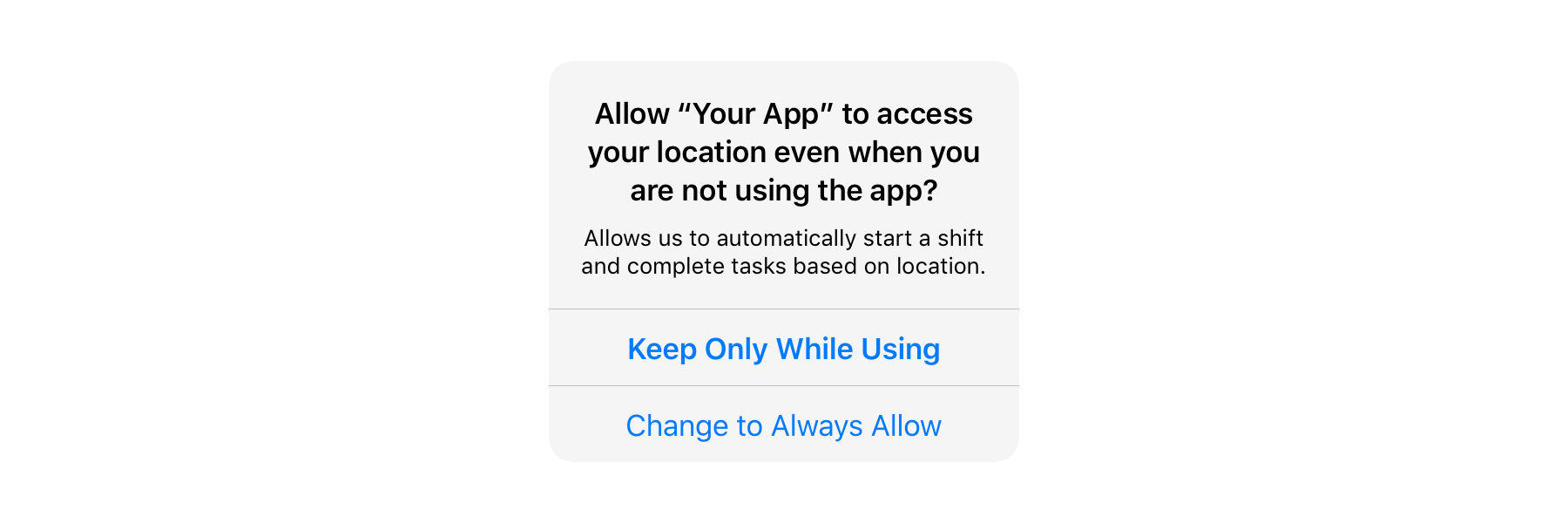In the image, there is a light gray rectangular dialog box containing a location access request. The main text is in black and reads: "Allow [Your App] to access your location even when you are not using the app?" Below this, in slightly smaller black text, it says, "Allow us to automatically start a shift and complete tasks based on location."

Two options are available underneath the request. The first option is "Keep Only While Using," written in blue with each word capitalized. The second option is "Change to Always Allow," also in blue and with each word capitalized. This dialog box is a typical pop-up that appears on a smartphone, asking the user for permission to access their location data even when the app is not actively in use.